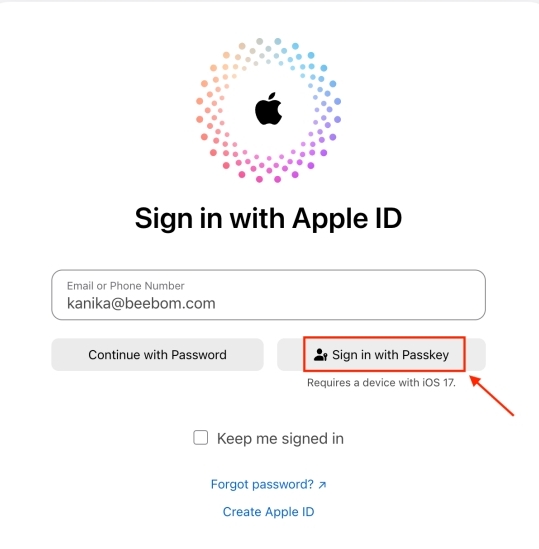This image is a detailed screenshot from an Apple device, potentially an iPhone or iPad, featuring the Apple ID sign-in interface. The background is predominantly white, and the iconic Apple logo is prominently displayed at the top. Central to the image is the text "Sign in with Apple ID" in bold black letters. Below this heading, there is a text field for entering the user's email address. Further down, there are two gray buttons: one labeled "Continue with Password" and the other labeled "Sign in with Passkey." A red arrow points specifically to the "Sign in with Passkey" button, suggesting that this screenshot might be used for instructional purposes, highlighting the option for emphasis. Beneath these buttons is a checkbox labeled "Keep me signed in." At the bottom, there are links for "Forgot password" and "Create an Apple ID," offering additional options for user account management.